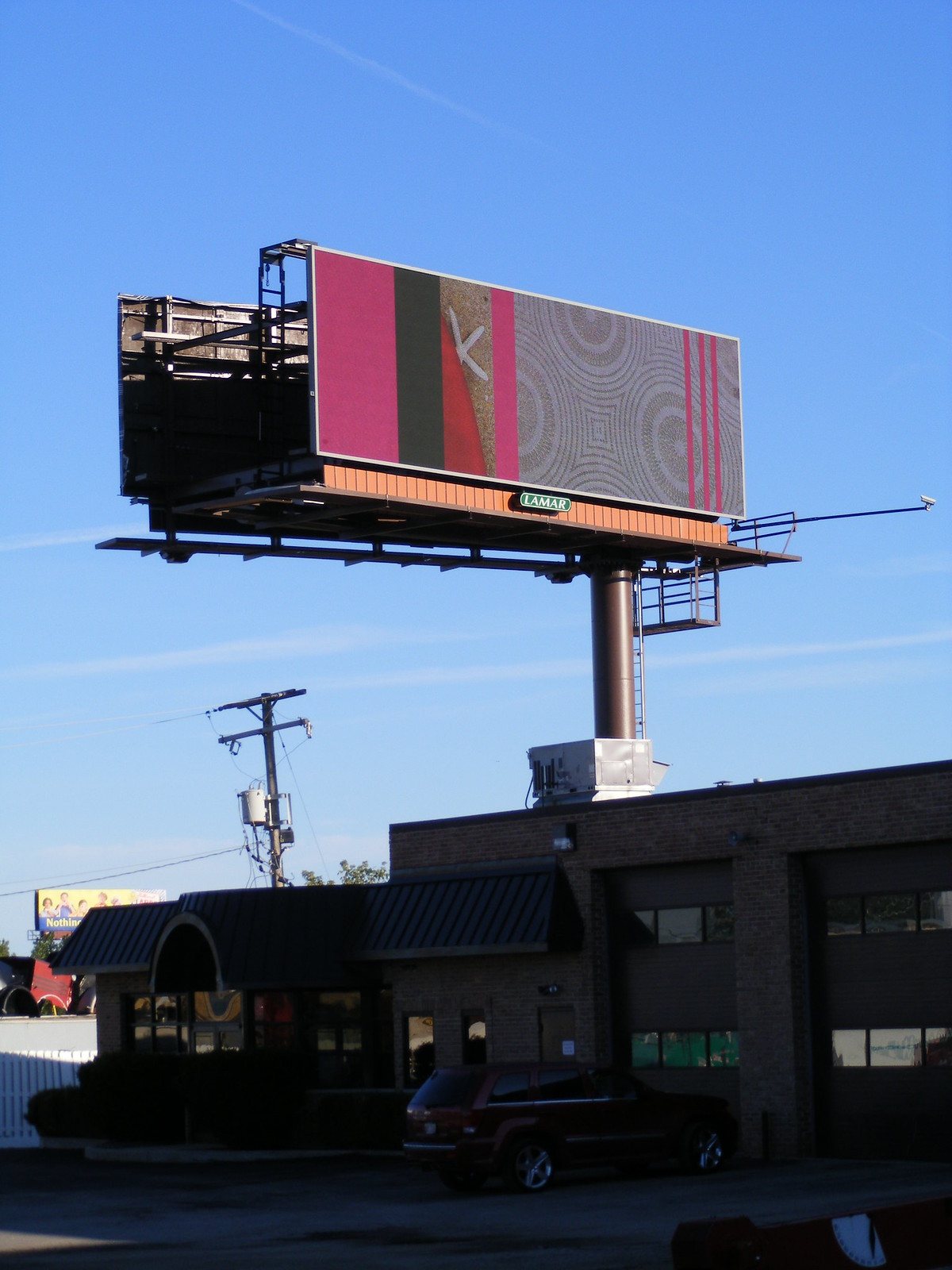On a serene, clear day, beneath a vivid blue sky with barely a cloud in sight, a captivating billboard stands prominently on the roof of a dark brick building. Mounted on a thick, brown pole, this dual-screen billboard features two displays—one facing the viewer and the other facing away. Below the screen, the name "Lamar" is boldly emblazoned. The screen presents an intriguing design with a sequence of colors and patterns: pink on the left, followed by a black stripe, a red object, a dried sand dollar or starfish in sand, another pink stripe, and circular patterns reminiscent of sand garden designs. Three pink lines distort part of the circular design on the right. 

A camera, mounted on a pole extending to the right of the billboard, keeps watch over the display. Access to the billboard is facilitated by a sturdy ladder that leads up to a maintenance platform. The building itself, constructed from dark bricks, features an aluminum awning over an arched doorway, flanked by shrubbery mostly obscured by shadows. 

In front of this building, a single dark SUV is parked, surrounded by a series of windows and doors. On the left side of the building, there are two windows, followed by a door flanked by more windows, and a solid, round door. The right side showcases a symmetrical arrangement of three windows on the top, three on the bottom, a break, then another set of three windows above and below.

In the background on the left, another distant billboard is vaguely visible. Though mostly unreadable, it appears yellow and possibly features five people. A power line runs along this side of the building, sporting a visible transformer, adding to the urban atmosphere of the scene.